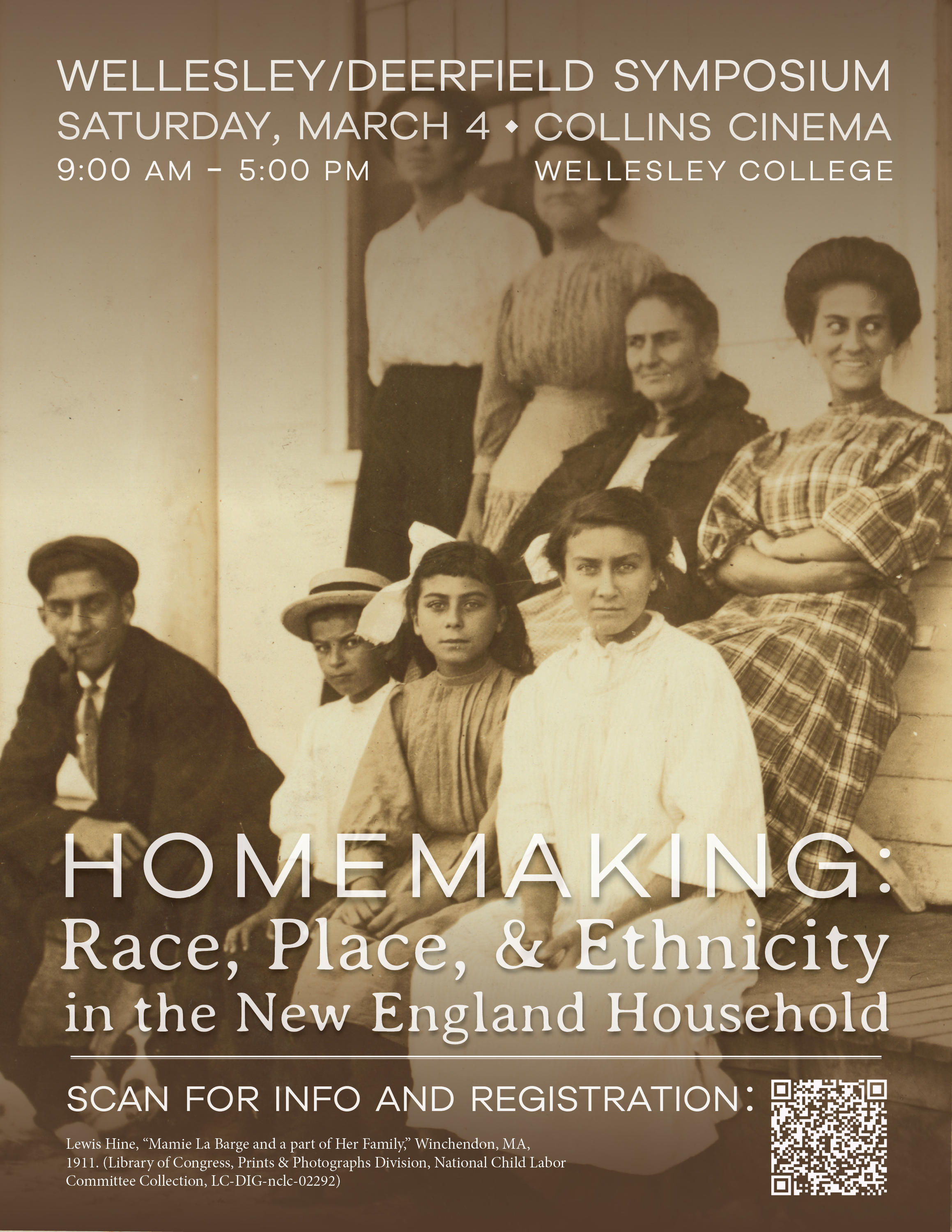Promotional image for the "Wellesley / Deerfield Symposium" captures a sepia-toned, vintage-style photograph of a group picture taken in Winchendon, Massachusetts in 1911. The photograph, sourced from the Library of Congress Prints and Photographs Division National Child Labor Committee Collection, shows a diverse group of men and women dressed in early 20th-century attire, with women in long dresses and men wearing suits and ties, seated on benches and steps in front of a building. The participants have medium skin tones and are arranged in two rows, with one row seated on the patio and the other standing behind.

At the top of the image, white text announces the event details: "Wellesley / Deerfield Symposium, Saturday March 4th, Collins Cinema, 9 a.m. to 5 p.m., Wellesley College." Beneath this, the symposium's theme is highlighted: "Homemaking, Race, Place, and Ethnicity in the New England Household." A QR code in the bottom right corner directs viewers to scan for information and registration. Additional text in the bottom left corner identifies the people in the photograph as "Lewis Hyde, Mamie Labarge, and part of her family."